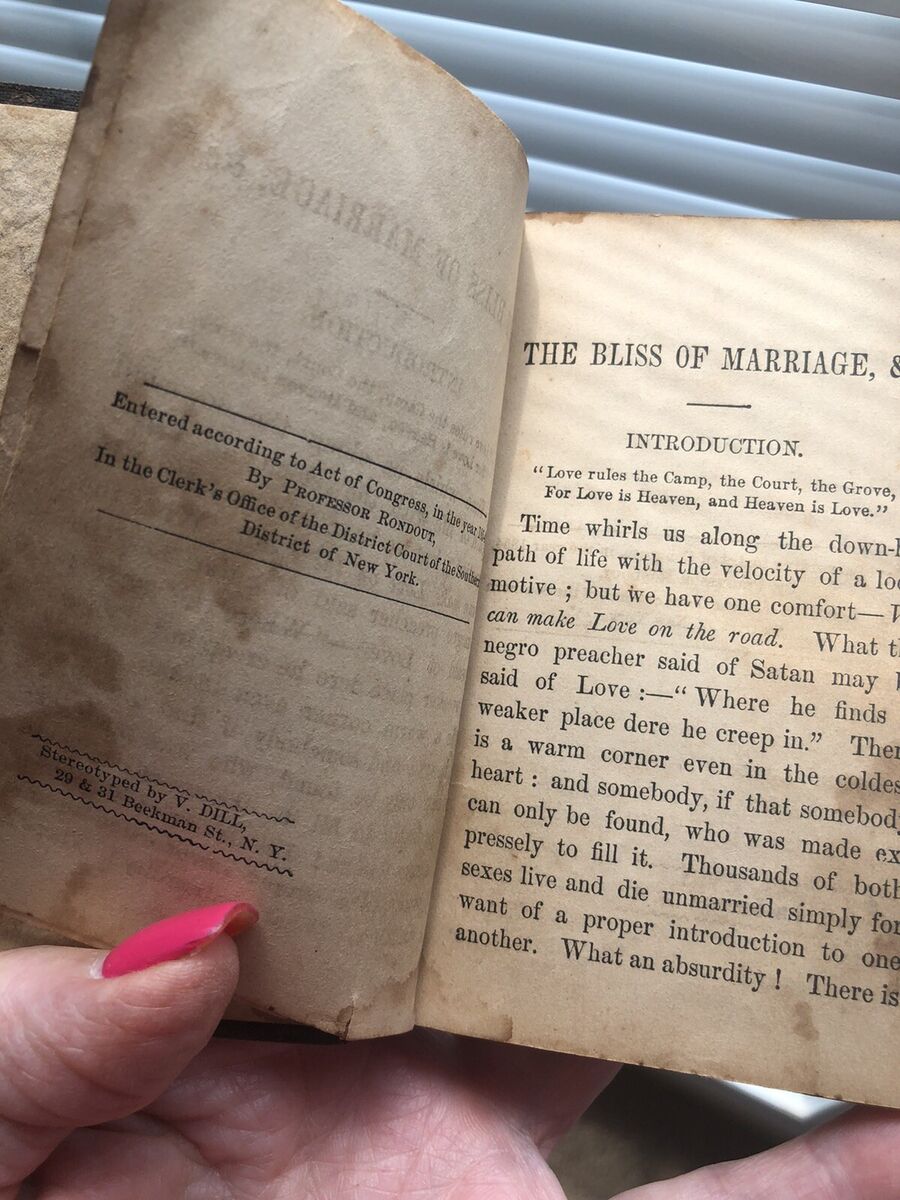In this color photograph, a woman with bright pink nail polish and what appear to be fake fingernails is holding open a very old, distressed book that shows significant wear and staining. The title on the first page is "The Bliss of Marriage," and it begins with an "Introduction." The left page contains some text, possibly handwritten notes, which include the barely readable statement, "Entered according to Act of Congress in the year [unreadable year], by Professor Ron Dowd in the Clerk's Office of the District Court of the Southern District of New York." Additionally, it mentions "Stereotyped by V. Dill, New York." This exquisitely detailed image captures the nostalgic essence of an ancient book intertwined with the modern touch of vibrant nail art.